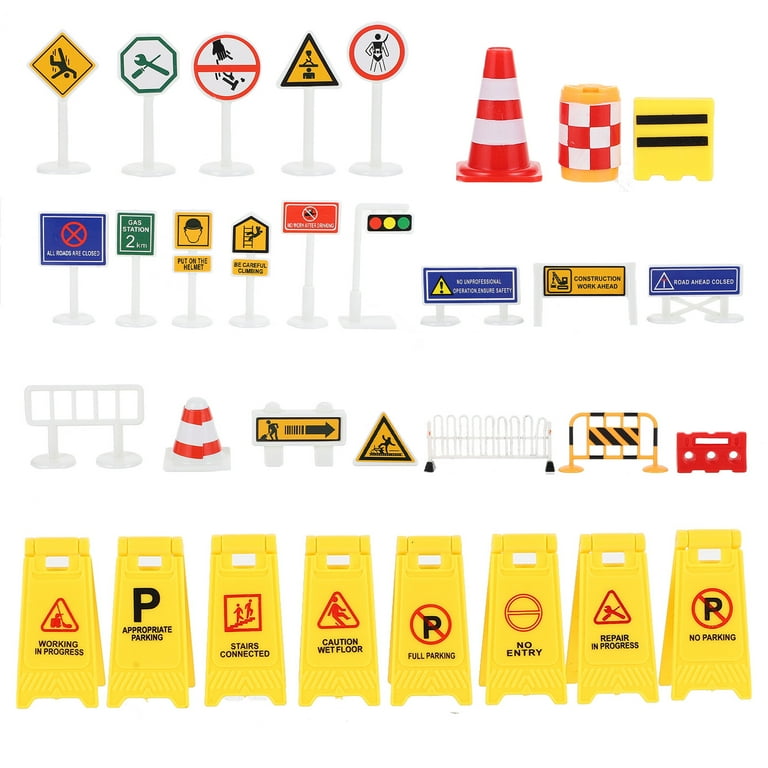The image displays a detailed collection of toy road and warning signs, set up in four rows from top to bottom, resembling what you might see in real-life traffic or construction zones but in miniature form, likely for a Lego game or similar. The top row features various signs, including a man slipping on a yellow "Slippery When Wet" sign, a green sign with a screwdriver and wrench, and a triangle sign with a yellow middle and black outline. There are also signs with a white background and a red line through them, indicating prohibitions, and a work sign with a figure in construction gear. Additional items in the collection are traffic cones and white-red striped barriers.

The second row continues with various colored signs – blue, green, yellow, red – indicating different road and traffic controls such as stop signs, signal lights, and directional arrows. Some of these items include signage for road closures and construction zones.

The third row features more practical signs like "Caution Wet Floor" and "Repair in Progress." There are also small gate structures, often used in parking spaces, painted white with wheels and markings. There's a red and white cone indicating no entry.

The bottom row consists primarily of yellow hazard signs, similar to those seen in hospitals or housekeeping scenarios, with messages like "Alternate Parking," "Full Parking," "No Entry," and "No Parking." This comprehensive collection provides a thorough representation of various road, hazard, and construction signs that are typically used to guide and inform.